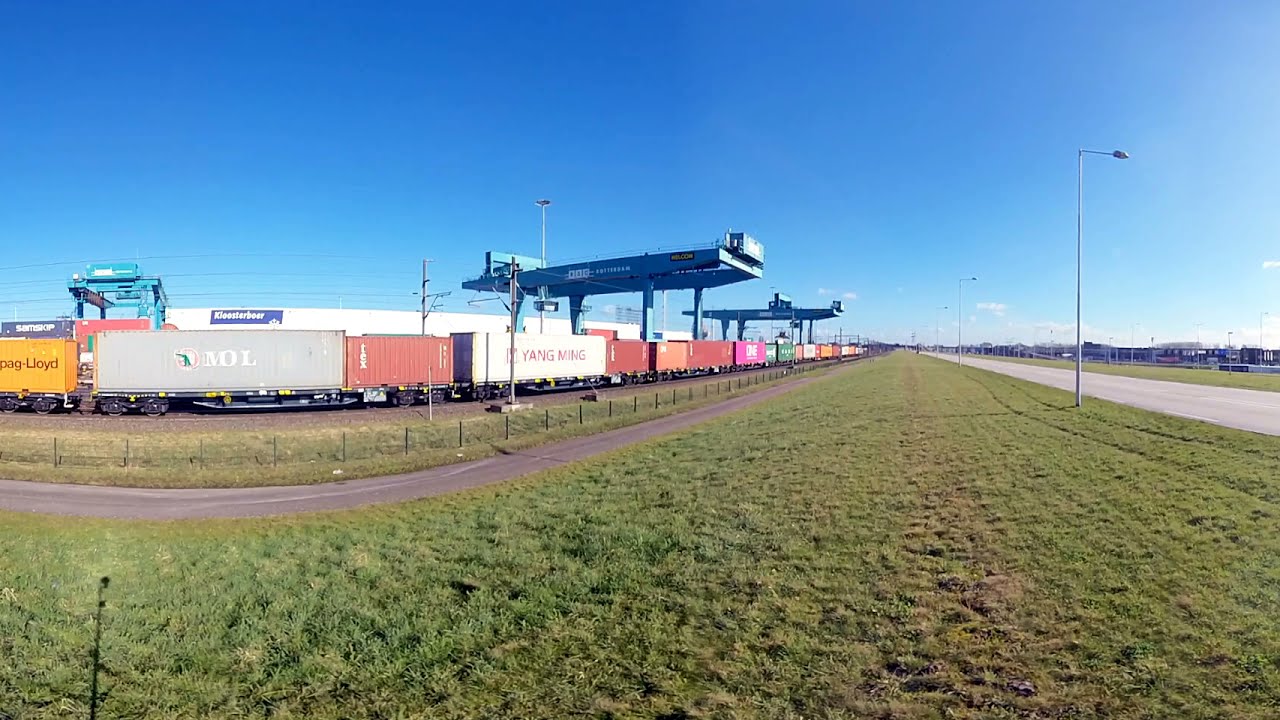This outdoor daytime image depicts a busy train depot extending from the left side of the frame toward the center and then continuing into the background. A long train with multicolored cars—yellow, gray, and red—marked with names like Yang Ming, MOL, and Lloyd, is visible. The train is partially covered by heavy-duty blue scaffoldings and overhead cranes, which are supported by robust metal beams.

To the right of the train, a green patch of grass is bordered by a tall, upright fence, beyond which a dark gray pathway or bike trail runs parallel. Further to the right is another strip of grass, featuring a mix of gray and yellow hues, adjacent to a light gray asphalt road. This road, stretching into the distance, is lined with street lamps that curve at the top to direct light downward.

In the background, you can see a clear blue sky with a few scattered white clouds, indicating a bright, sunny day. The shadows cast by the streetlights suggest that the sun is positioned on the right side of the image. Buildings are faintly visible in the far distance on the right side, adding depth to this scene of industrial and natural elements combined.